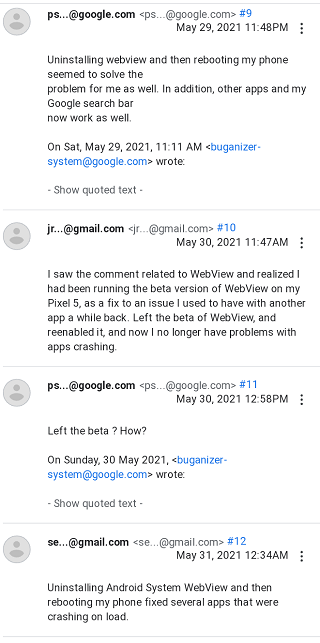This detailed caption describes a screenshot taken from a phone, specifically from a comment section related to troubleshooting an issue:

---

The screenshot showcases a detailed comment section from a mobile phone, likely addressing a troubleshooting forum. The first comment, timestamped May 29, 2021, at 11:48 p.m., is from a user with the email prefix 'ps' at google.com. They explained that uninstalling WebView and rebooting their phone successfully resolved their issue. They also mentioned that other apps and Google Search started functioning properly post-troubleshooting. In response, the system acknowledged their comment at 9:11 a.m.

Further down, another comment highlights a user who saw a related suggestion about WebView. They mentioned that they had been using the beta version and decided to leave the beta on Sunday. The process they followed is also briefly described, including uninstalling the Android System WebView.

---

This caption captures the essence of the screenshot, providing a clear and descriptive summary of the conversations and context within the image.